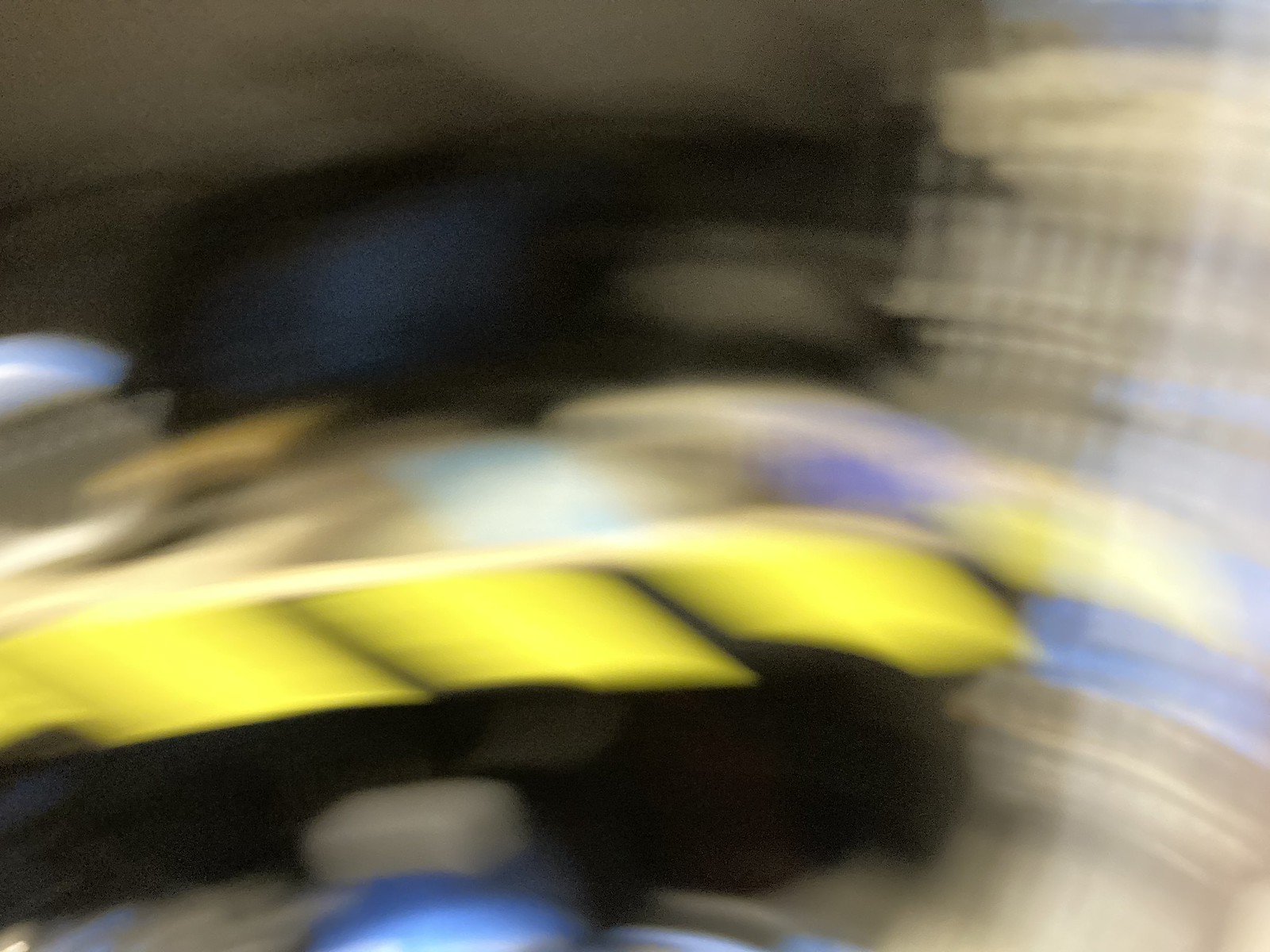This photograph teeters on the edge of the abstract, captured with a long exposure technique that imbues it with the fluid qualities of a painting. The upper portion is a swirling vortex of soft greys and blacks that merge and separate like tense brush strokes. Hints of blue and yellow peek through the monochromatic haze, suggesting a hidden vibrancy. Below this, streaks of brown and blue cascade in smudged, light-colored trails, giving the image a sense of motion and depth. Interspersed amidst these softer hues are three bold flashes of yellow, punctuating the composition with luminous energy. A large, imposing black rectangle sits solidly beneath these yellow bursts, providing a stark contrast to the fluid background. Amidst all of this, a curious shape emerges: a grey button-like form centered on a blue disc, anchoring the visual chaos with an element of structure. Whether it's an abstract painting, a computer-generated design, or a fast-moving photograph of real objects, this image captivates with its intriguing blend of color, texture, and form.